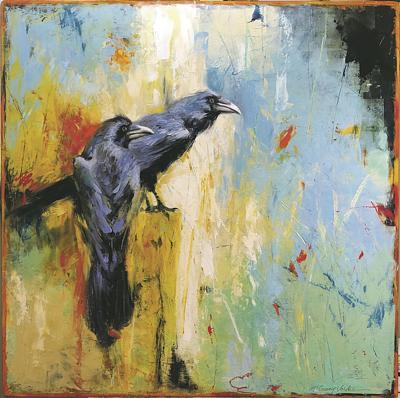This vibrant oil painting features two blackbirds, likely ravens, perched awkwardly on a bright yellow ledge. Both birds are staring towards the right, captivated by something outside the frame. The background is a dynamic mix of colors: the right side is dominated by splattered patterns of blue, yellow, red, and darker blue, culminating in a pure black corner at the top right. The left side showcases the two ravens against a yellow field, with the top left corner mirroring the blue hues from the right side. Red birds and small red, flower-like dots add complexity, while splashes of green and white accentuate the scene. Despite the chaotic, graffiti-esque backdrop, the painting’s blend of light and color suggests the sun is illuminating the birds. No text or signature reveals the artist, and other than the vividly rendered avian subjects, the painting is devoid of additional objects.